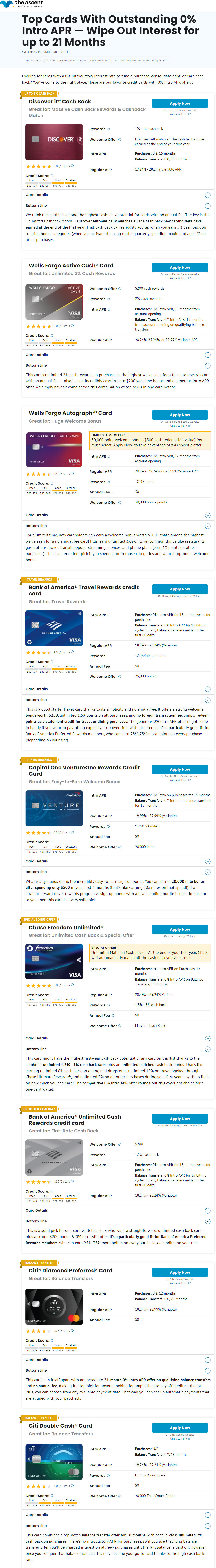The image features a white background with a blue element in the upper left corner. This section contains very small, illegible black text. Below this, there is a gray background with readable black text stating, "Top Cards with outstanding 6% intro APR wipes out interest for 21 months." This indicates that the image is about credit card offers.

On the left side of the image, there is a vertical list of various credit cards, each card accompanied by a significant amount of text. These cards include:

1. A black credit card
2. A silver credit card
3. Another black credit card
4. A blue credit card
5. A blue credit card with white text
6. Another black credit card, potentially a darker blue
7. A gray credit card
8. A light gray credit card
9. Another black credit card
10. A darker gray credit card

To the right of each card, there is a large button, either white or blue with white text, likely intended to direct users to the respective company's website to apply for that specific credit card.

The remainder of the image contains very fine print and other details that are unreadable.